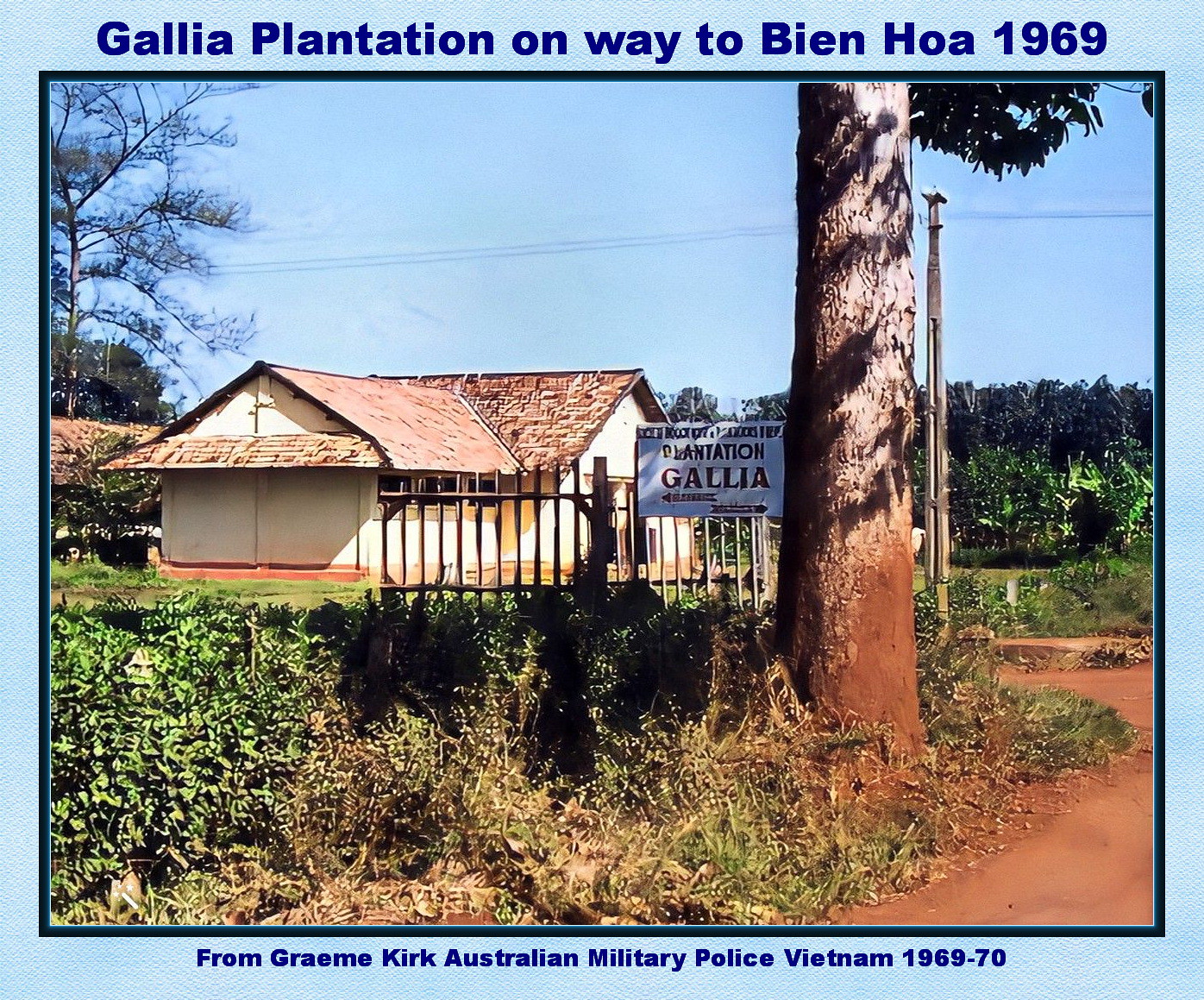This photograph, set against a light blue background, depicts the Gallia Plantation en route to Bien Hoa, Vietnam, captured in 1969. The top of the image bears a dark blue inscription: "Gallia Plantation on way to Bien Hoa 1969." The bottom reads, also in dark blue: "from Graham Kirk, Australian Military Police, Vietnam, 1969-1970." Central to the composition is the plantation itself, framed in black. The scene includes a light tan building with a thatched or brown wooden roof, set amidst a verdant landscape of trees and shrubbery under a clear blue sky. A large tree stands prominently in the front, with a partial fence and a dirt road leading to the building. The fence features a sign reading "Plantation Gallia" with directional arrows pointing left and right. Additionally, a tall tree is visible on the far left of the image, with a power line running horizontally across the middle, above the house. This poignant image, likely captured by Graham Kirk during his service in the Australian Military Police, offers a glimpse into the serene yet historically significant locale during the Vietnam War.